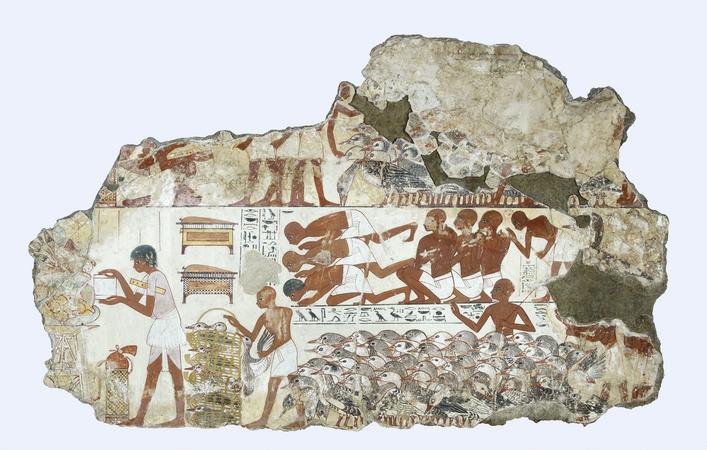This is an image of an ancient Egyptian artifact, possibly a broken piece of wall or pottery. The artifact features a group of dark-skinned figures, which include both men and one woman. The men, who are depicted with no hair, are shirtless and wear white garments wrapped around their lower bodies. Some men are bowed down as if in prayer or work, while one man holds birds. In contrast, the woman, who has dark hair and a ruler under her arm, is fully clothed in a skirt and shirt. Several birds, likely geese, are gathered in the foreground, some being enclosed in cages or containers. The artifact has jagged, broken edges and shows visible signs of age or damage, giving it an authentic ancient appearance. The background of the image is a light blue color, drawing attention to the artifact, which includes hieroglyphs and is depicted in earthy tones of tan, brown, and hints of green. The square image, devoid of any border, appears to have been carefully staged and captured using natural light.